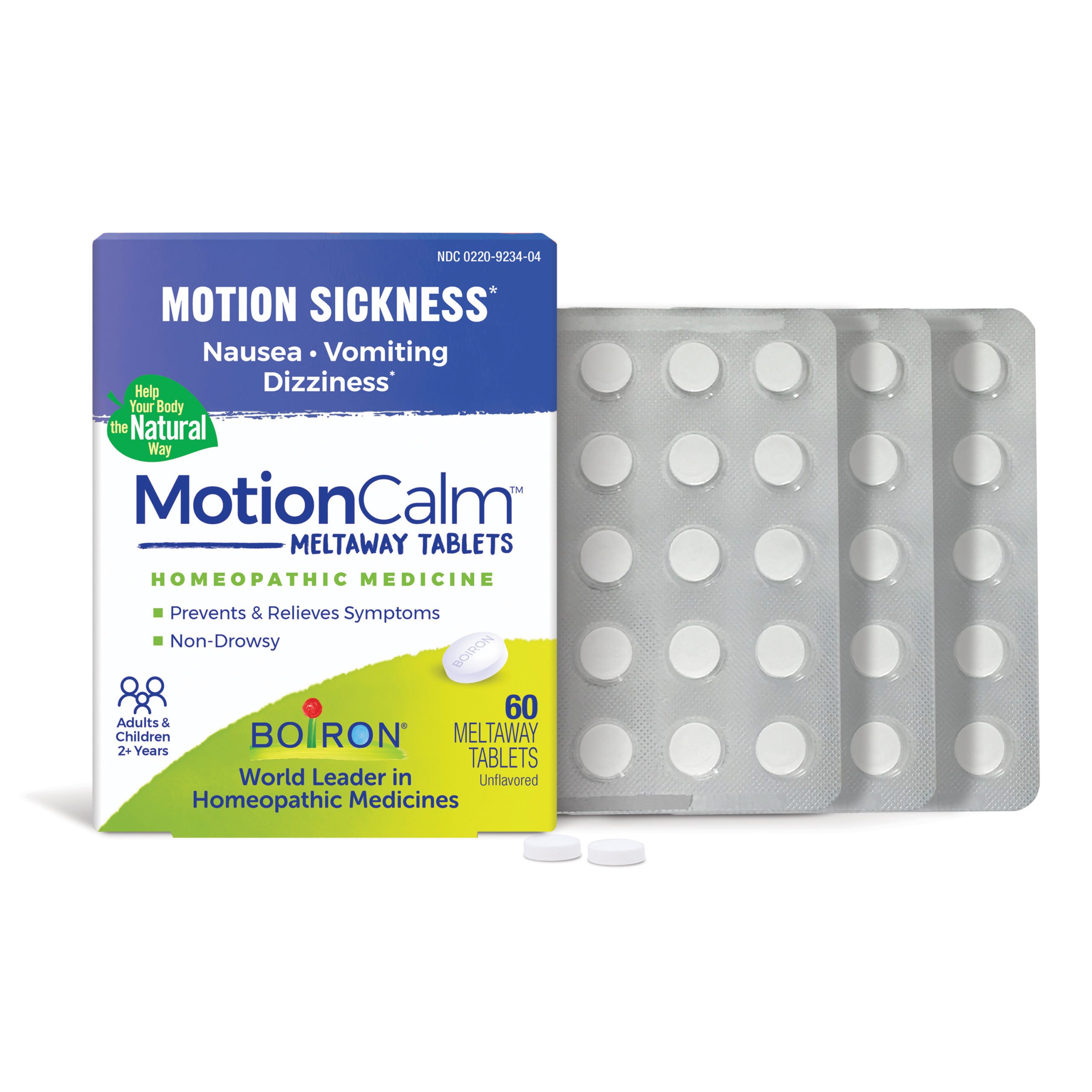The promotional color photograph showcases Boiron’s Motion Calm Homeopathic Medicine against a white background. On the left, the blue, white, and yellow box prominently displays its purpose with text that reads "motion sickness, nausea, vomiting, dizziness" in white lettering on the blue section. A small green leaf icon with the phrase "help your body the natural way" adds a natural remedy touch. Below in the white section, "Motion Calm" is highlighted along with descriptors like "melt-away tablets" and "homeopathic medicine" labeled in green text. The yellow section on the lower portion of the box provides additional product details and an image of one of the tablets. To the right of the box, three silver blister packs expose the white, circular tablets through clear viewports. Additionally, two tablets are placed on the white surface in front of the blister packs, emphasizing the non-drowsy formula that helps prevent and relieve motion sickness symptoms naturally.